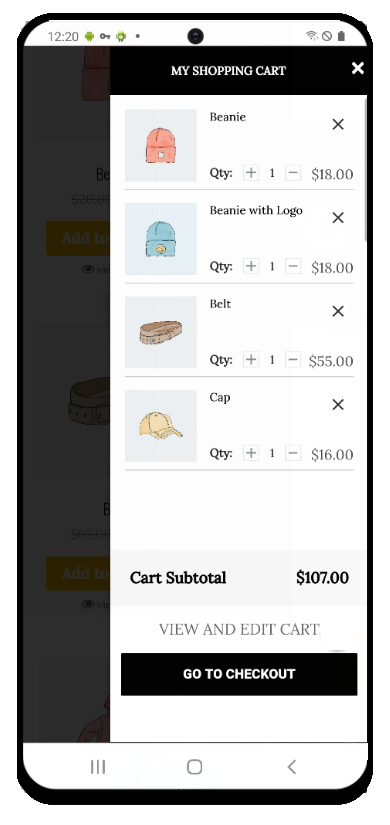Screenshot of a phone mock-up displaying a shopping cart on a website app. The top of the screen features a black bar with the text "My Shopping Cart" in white, accompanied by a white X button on the right side for closing the cart. Below this header, there is a detailed list of items currently in the shopping cart. Each item on the list includes a thumbnail image on the left, the item title in the center, and an X button for removal on the right. Directly beneath each item title, there's an interface for adjusting the quantity, including a plus button to increase the quantity, a numerical display showing the current quantity (default at one), a minus button to decrease the quantity, and the price of the item.

The items in the cart are as follows:
1. Beanie - $18
2. Beanie Logo - $18
3. Belt - $55
4. Cap - $16

At the bottom of the list, the cart subtotal is displayed, summarizing the total cost of items before tax and shipping. Below the subtotal, there is an option labeled "View and Edit Cart" for further modifications. Finally, at the very bottom, there is a prominent black button labeled "Go to Checkout" to proceed with the purchase.